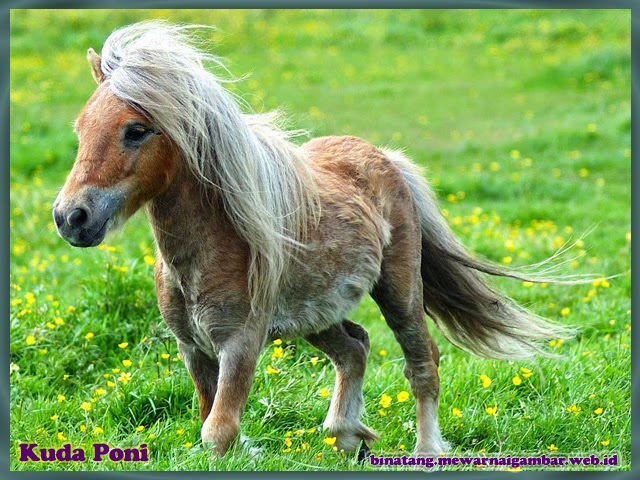In this close-up image, a cute miniature pony is depicted amidst a lush field of green grass dotted with yellow flowers, possibly dandelions. The pony, slightly positioned to the left of the center, features a long flowing mane and a tail that appears to be blowing in the wind, indicating a slightly breezy day. Its white legs and black nose add to the charming details of this small, adorable creature. The primary colors in the image include shades of green, yellow, brown, white, and pops of purple from the text overlays. In the lower left corner, in purple letters, it reads, "Coup de Pony," spelled as "K-U-P-O-N-Y." Meanwhile, the lower right corner displays a web address in purple: "B-I-N-A-T-A-N-G dot M-E-W-A-R-N-A-I-G-M-B-A-R dot W-E-B dot I-D." There are no other elements in the picture, which focuses solely on the pony in an outdoor, natural setting, emphasizing its serene and picturesque surroundings. The sky is not visible in the image, as the camera angle points slightly downward.